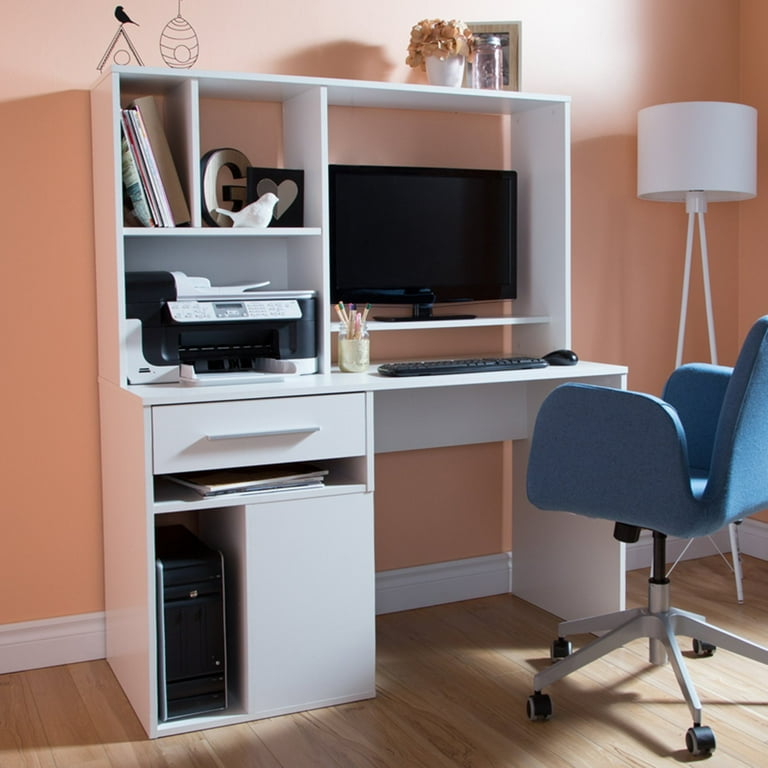The image captures a home office bathed in daytime light filtering through windows. The focal point is a white computer desk adorned with various items and set against a peach-colored wall, accentuated with a white border. Light-colored wooden floors add warmth to the indoor setting.

To the right in the corner stands a tall, white lampshade. A blue, wheeled chair resembling a stool is positioned in front of the desk. The desk itself, predominantly white, features multiple shelves and compartments. A computer monitor is situated on one of the shelves with a keyboard and mouse directly below it. On the left side of the desk, the computer tower is housed within a vertical compartment, alongside a small closed drawer. 

On the shelves above, there is a black printer to the left. To the right of the printer is a section holding books, a white bird figurine, and another small G-shaped figurine with a heart design. Above these, at the top of the unit, there are decorative elements including a small vase with artificial orange flowers, a framed photo, and a glass bottle. The left-most shelf also displays some artwork stickers featuring a birdhouse, a bird, and a beehive.

The meticulous arrangement of the home office—a blend of technology, books, and decorative items—creates a well-organized and aesthetically pleasing workspace.